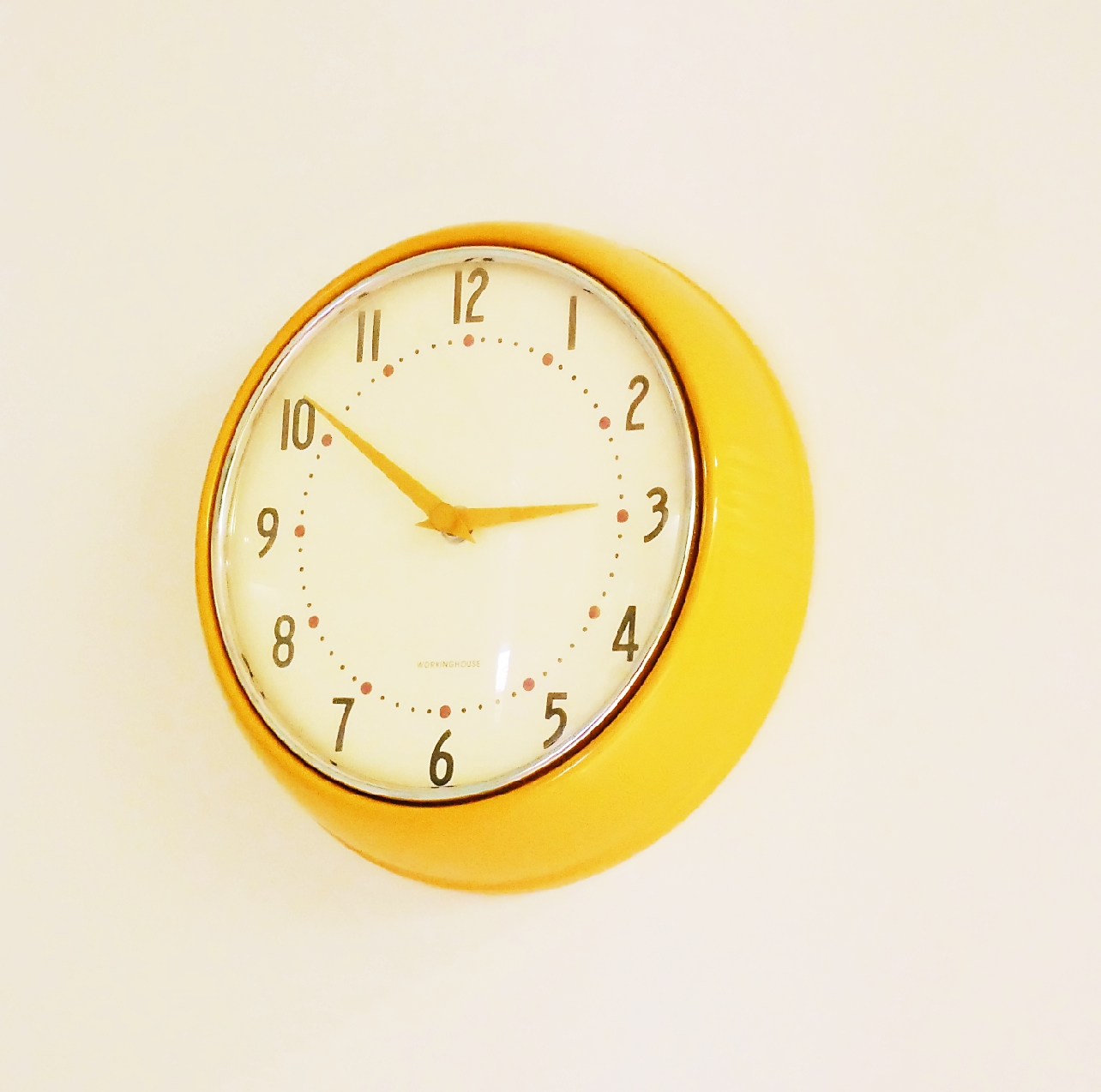This image features a stylish, vintage-inspired wall clock with a distinctive yellow ceramic frame. The clock, mounted on an off-white, possibly eggshell-toned wall, showcases a round, 3D appearance. The clock face is white and protected by a glass cover, which adds a subtle shine. It includes brown numbers in a slender, somewhat Art Deco font, arranged in the traditional 1 to 12 format. The hour indicators are marked by black dots, except for the red dot at the standard hour positions. Both the hour and minute hands, also yellow, point respectively to just above 10 and around 3:50. At the lower part of the clock face, there is some writing that is not easily discernible, contributing to the clock’s unique and intriguing aesthetic.